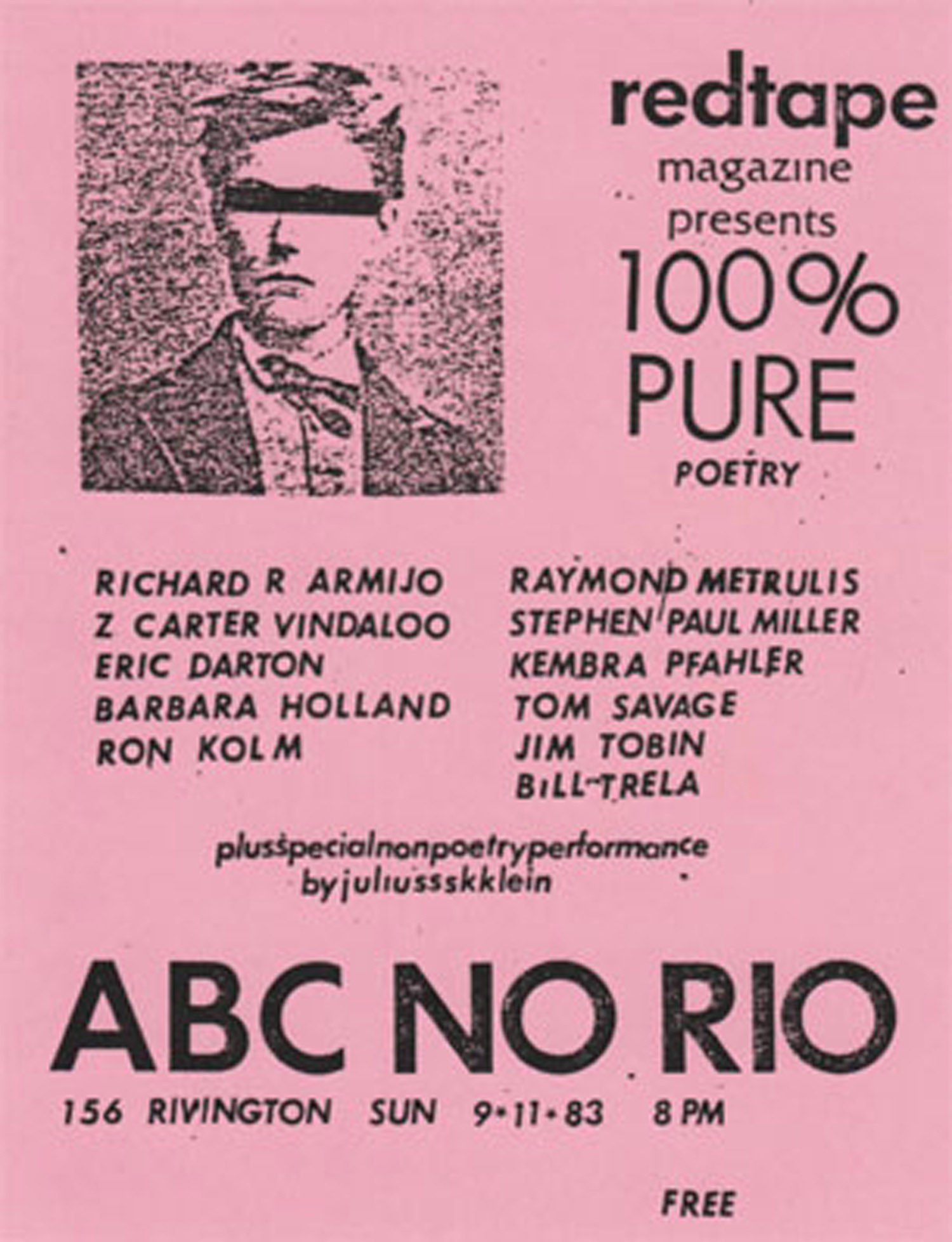This is a vintage promotional poster, likely from around September 11th, 1983, issued by Red Tape Magazine for an event titled "100% Pure Poetry". The event is advertised on a pink, possibly medium lilac, background with a black and white, pixelated image of a man in an old-fashioned suit, perhaps from the late 1800s or early 1900s. His short hair and the black rectangular bar concealing his eyes give the image a mysterious, staticky appearance. The poster lists performers including Richard R. Armijo, Z. Carter Vindaloo, Eric Darnton, Barbara Holland, Ron Colm, Raymond Metroulis, Stephen Paul Miller, Kembra Pathaler, Tom Savage, Jim Tobin, and Bill Trella. Additionally, it mentions a special non-poetry performance by Jules Scaline. The event is to be held at ABC No Rio, located at 156 Rivington, on Sunday, September 11, 1983, at 8 p.m., and entry is free.